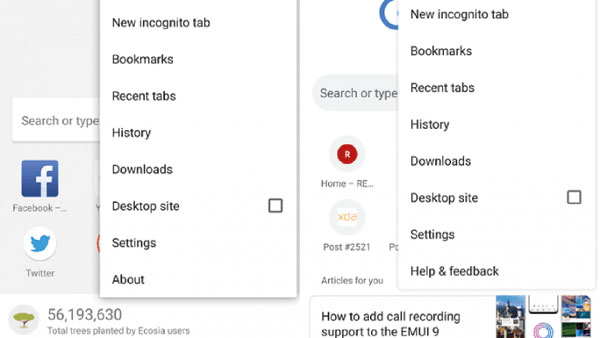The image comprises a series of overlapping screenshots. On the left side of the image, there is a gray and white interface with a search box labeled "Search or type". Nearby are the icons of various social media platforms, including the white and blue Facebook logo and the blue and white Twitter logo. Adjacent to these is a pop-up menu with black text on a white background, listing options such as "New incognito tab," "Bookmarks," "Recent tabs," "History," "Downloads," "Desktop," "Site settings," and "About". At the bottom of this section, there is a green icon resembling a bird, accompanied by a statistic reading "56,193,630 total trees planted by ECOZA users."

On the right side of the image, another background shows a website interface, featuring a search box and several shortcut icons, including a red and white one and an orange and white one. A similar pop-up menu appears here too, with options like "New incognito tab," "Bookmarks," "Recent tabs," "History," "Downloads," "Desktop," "Site settings," "Help," and "Feedback." At the bottom, black text reads "How to add call recording support to the EMUI 9" next to a photograph resembling an old iPod with a circular controller, a white screen, and a mix of purple and blue colors. Behind this central image, there is a series of other images: one predominantly blue, another tan, one with purple, blue, and orange hues, and a partial image of a person towards the bottom. The rest of the details in the image are relatively mundane.